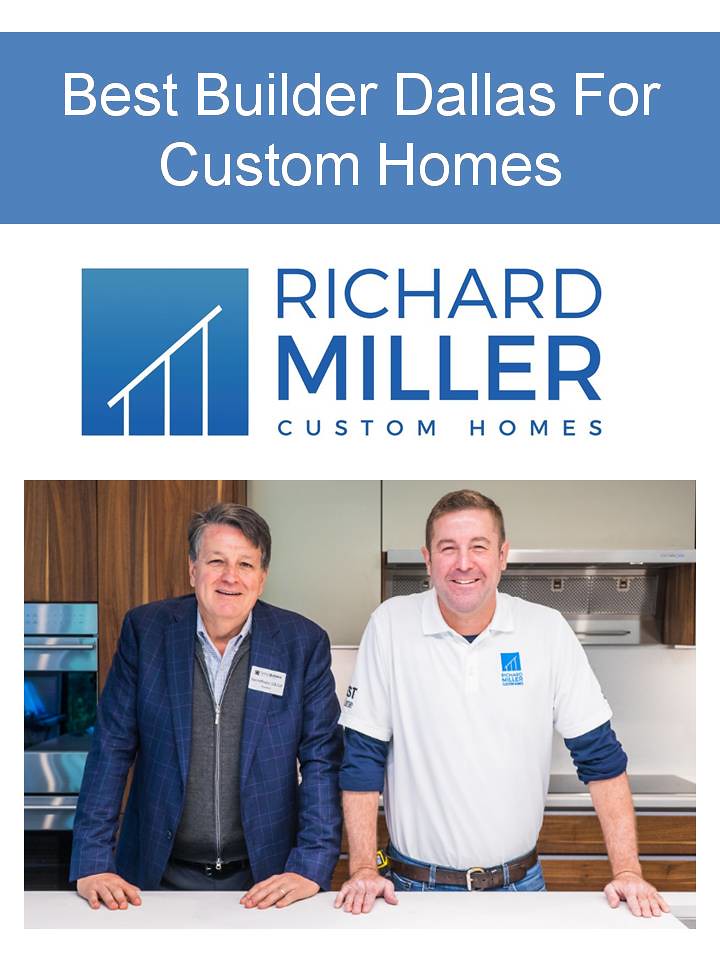The image appears to be an advertisement for a custom home building company. At the top, a blue banner displays the text "Best Builder Dallas for Custom Homes" in white. Beneath the banner, the name "Richard Miller Custom Homes" is prominently featured in blue with "Miller" emboldened. To the right of the text, there is a blue square with a simplistic white house logo and the words "Custom Homes."

The photo shows two men standing side-by-side in a kitchen. The man on the left is slightly older, appears to be in his 50s, has short hair that is slightly balding, and is smiling. He wears a blue suit jacket over a gray zip-up sweater and a light blue button-up shirt, paired with blue jeans. He is also seen wearing a name tag. The man on the right, also seemingly in his 50s, has short hair and is dressed in a white polo shirt over a dark blue long-sleeve shirt with rolled-up sleeves. He is wearing blue jeans and a visible brown belt. His white shirt bears the company logo.

The kitchen setting behind them includes brown wooden cabinets, a white countertop, a range, and an oven, adding context to their expertise in custom home building.